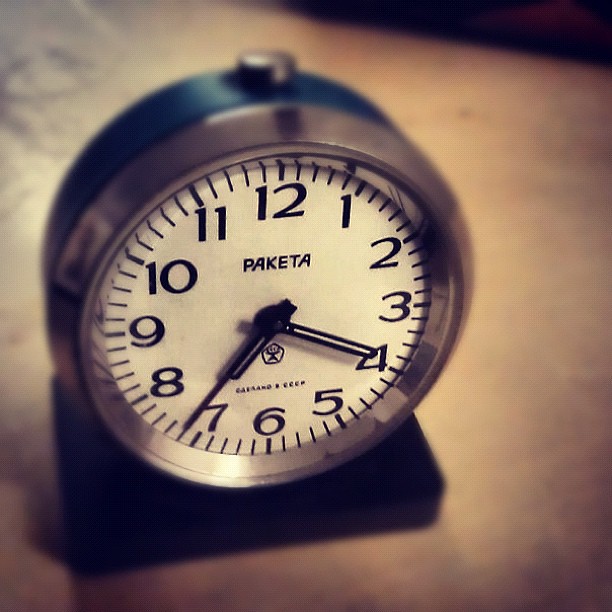This photograph features a vintage-style clock prominently displayed on a counter, which appears to be white or off-white in color. The image adopts a grayish, almost monochromatic tone, reminiscent of black-and-white photography. The clock, positioned towards the bottom left corner of the frame, has a back surface that is black with a noticeable silver button. The front of the clock showcases a sleek silver bezel encircling its face. It stands securely on a small square base, colored black to match the back. 

The clock's face is white, providing a stark contrast to its black numerals. Notably, the number 12 is replaced with the brand name "P-A-K-E-T-A." The clock features black hands, which are currently indicating the time as 7:20. The overall composition of the image, combined with its subdued color palette, draws attention to the intricate details and classic design of the timepiece.